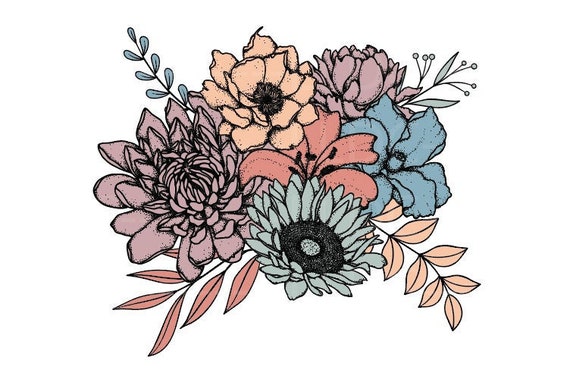The image depicts a vibrant, detailed illustration of a floral bouquet, set against a solid white background that dominates the composition. The flowers are beautifully clustered together, outlined in black, and each bloom is filled with solid, vivid colors. On the left side of the bouquet, the largest flower is a rich purple, with a blue flower positioned right below it. Centrally located is a striking red flower, flanked by more blossoms—another purple flower at the top, accompanied by a yellow flower near it, and another blue flower on the right side. The artwork also features twigs with leaves in dynamic hues of orange and blue, enhancing the bouquet's lively appearance. This meticulously colored, poster-like digital art captures the essence of floral illustration with its simple yet intricate design.